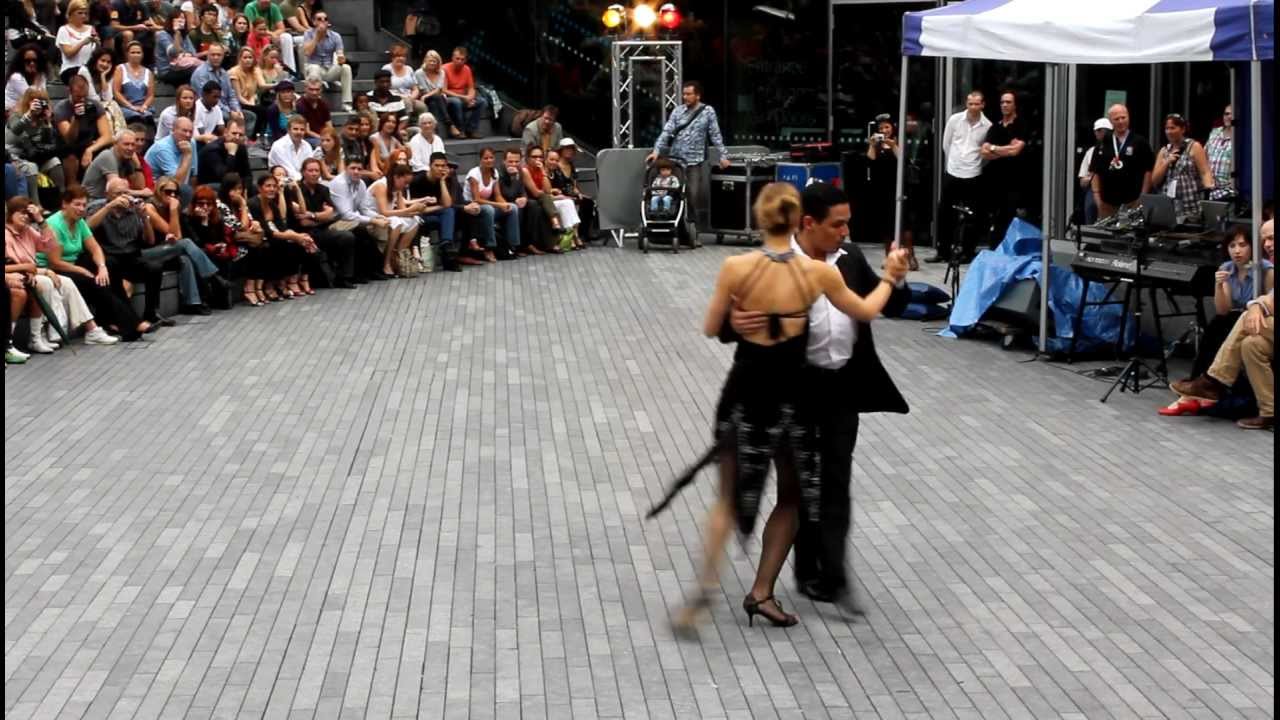This image captures an elegant moment of a couple dancing indoors, slightly right of center in the photograph. The woman, dressed in a striking black and white backless dress adorned with a floral print, has her blonde hair pulled into a bun. Her black shoes are visible, though her swift movement causes her left leg and the bottom of her dress to blur. She holds the man's hand aloft with her right hand. The man, with short black hair, is dressed in a sophisticated ensemble—a white button-up shirt beneath an unbuttoned black jacket and black pants, complete with black dancing shoes. His head is turned to the right as he places his spare hand on the woman's upper back. They dance on a light gray wooden floor that spans the width of the image. 

In the upper parts of the photo, a lively scene unfolds: to the right is a tent structure housing black equipment and several seated individuals, alongside a crowd standing beyond it. On the left side, a person with a baby stroller stands in front of some more equipment, near a metal arch adorned with lights. Further left, a stadium-like seating area is visible, with the first row completely occupied and several additional rows filled with spectators. The precision and style of the dancers suggest they are professionals, performing in front of an attentive audience.